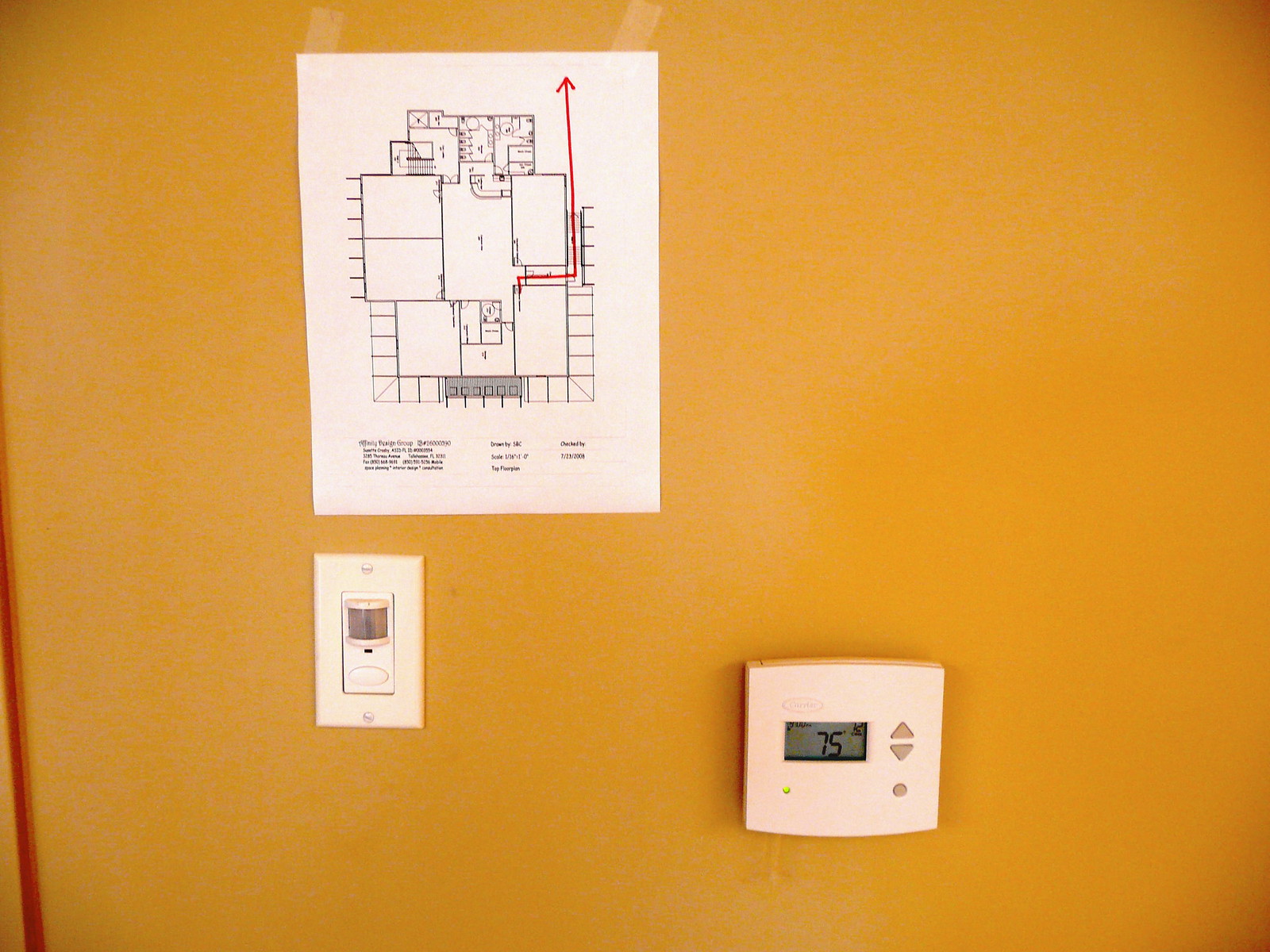The photograph captures an orange, possibly ochre-colored wall featuring several key objects. Centrally positioned is a digital thermostat, equipped with two buttons indicated by up and down arrows, currently set to 75 degrees Fahrenheit. Adjacent to the thermostat is a motion sensor with a single button, likely designed to activate lighting automatically when motion is detected. Above these devices, a detailed fire evacuation map is mounted on the wall. The map includes a prominent red arrow, denoting the viewer's current location, and outlines the emergency exit route, instructing individuals to turn right and then take the first left to safely exit the building in case of a fire.